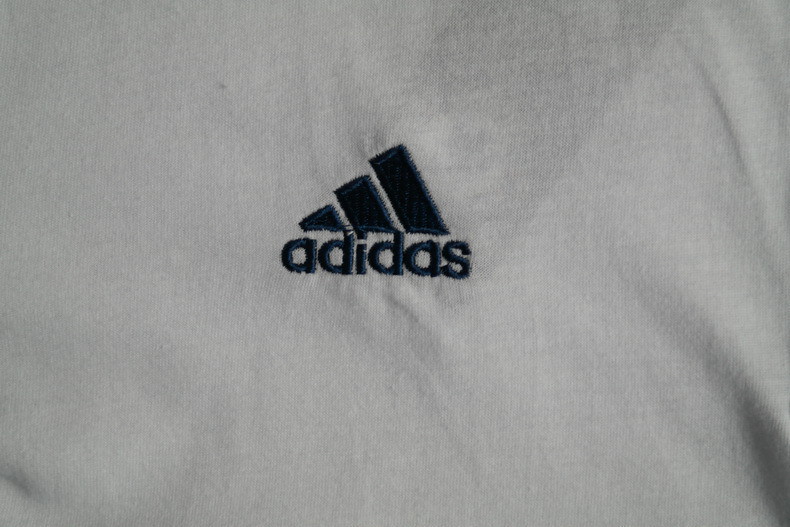This image provides a close-up view of a cotton garment, likely a t-shirt or sweatshirt, prominently featuring the Adidas logo. The Adidas name, "A-D-I-D-A-S," is displayed in a dark blue hue, providing a striking contrast against the pristine white fabric of the garment. The iconic Adidas symbol, a triangle oriented sideways and segmented into three distinct sections, sits above the brand name. The fabric appears tightly knit, highlighting the garment's high-quality construction. Noteworthy is a minor imperfection below the 'Adidas' name where the fabric shows a slight indentation and a small area on the right side that is slightly bunched up.